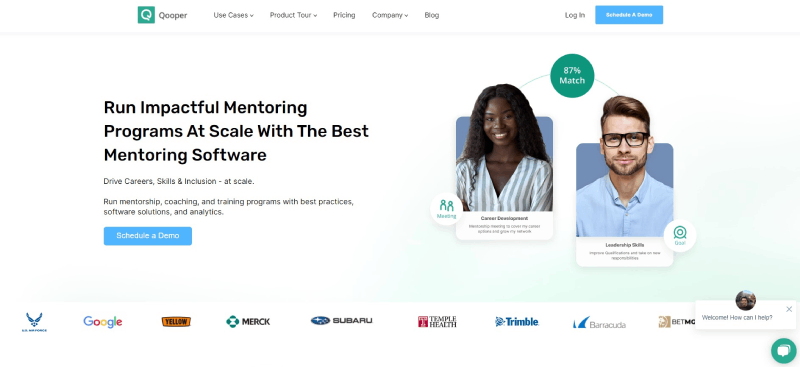The image showcases a website with a prominent header that is somewhat unclear but seems to include the letters "Q-E-O-P-E-R" or possibly "Q-O-O." On the top left, a green box with the letter "Q" is visible. The navigation menu includes links to "Use Cases," "Product," "Tour," "Pricing," "Company," and "Blog." Additionally, there are options to "Log In" or "Subscribe" within a blue box, although the text is too small to decipher clearly.

In the main section of the website, a bold headline states, "Run impactful mentoring programs at scale with the best mentoring software." Below this, there is a photograph featuring a Black woman and a White man, along with a caption indicating an 87% match, followed by brief descriptions about each individual. The text further promotes the software's ability to "drive career skills and inclusion at scale," and mentions that it supports running "membership, coaching, and training programs" with best practices, software solutions, and analytics. 

A blue "Schedule a Demo" button is prominently displayed beneath this content. The section further down lists supporters including "Merrick," "Google," a logo featuring an eagle, an orange box logo, "Triple Health," "Trimple," and another logo with an eagle and a brown image.

On the bottom right, a chat box is visible with a message saying, "Welcome, how can I help?" Next to it, a green circle with a white image can be seen.